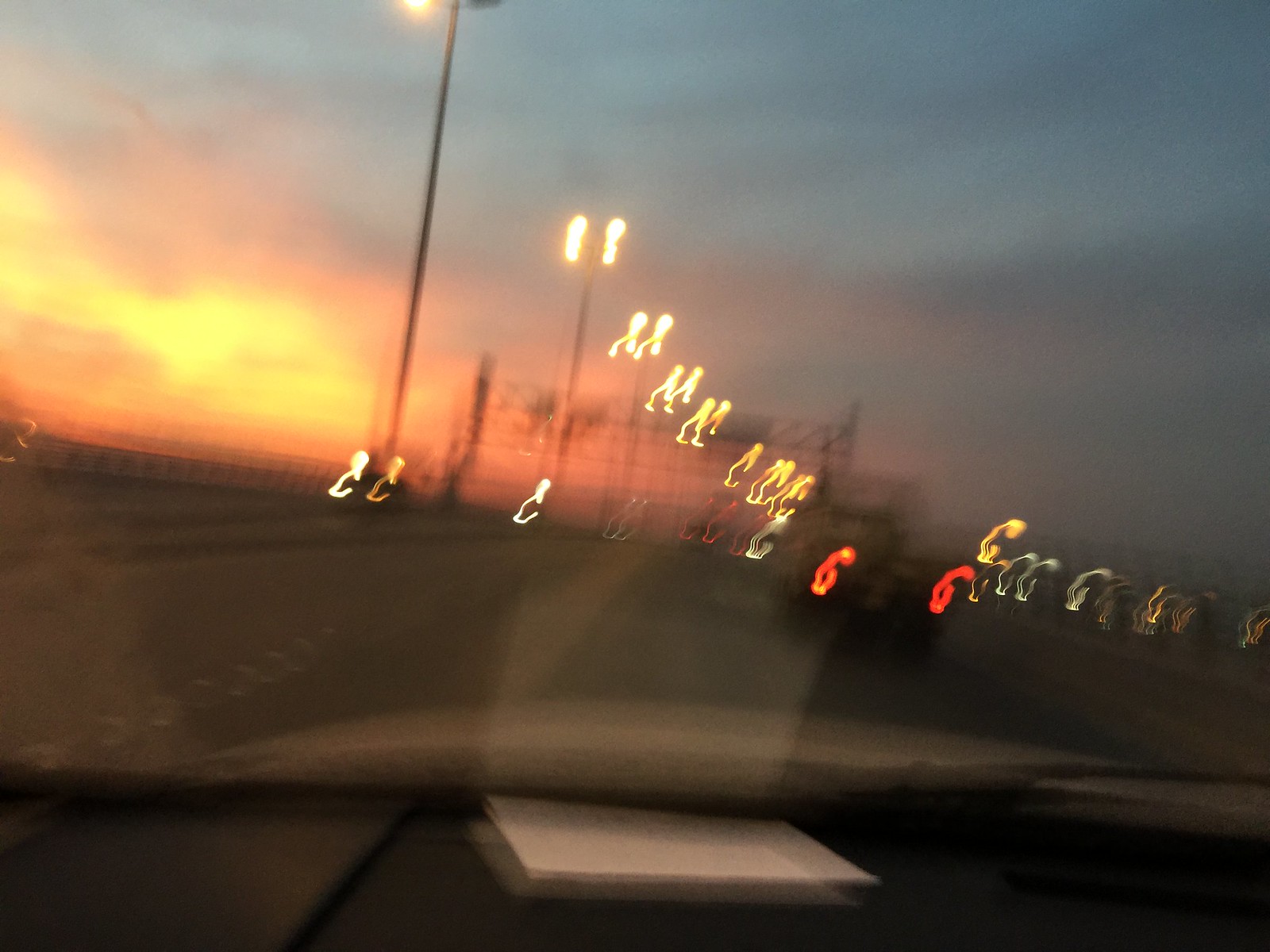A blurry, low-resolution image captured from inside a vehicle showcases an outdoor scene at twilight. The sky is a gradient, transitioning from a warm yellow and orange hue in the top left corner to a cooler blue and gray-black shade in the top right. Several cars are visible on the road, their headlights and taillights distinguishable amidst the haze. Streetlights overhead illuminate the scene with a stark white glow, piercing through the overall fuzziness of the image.